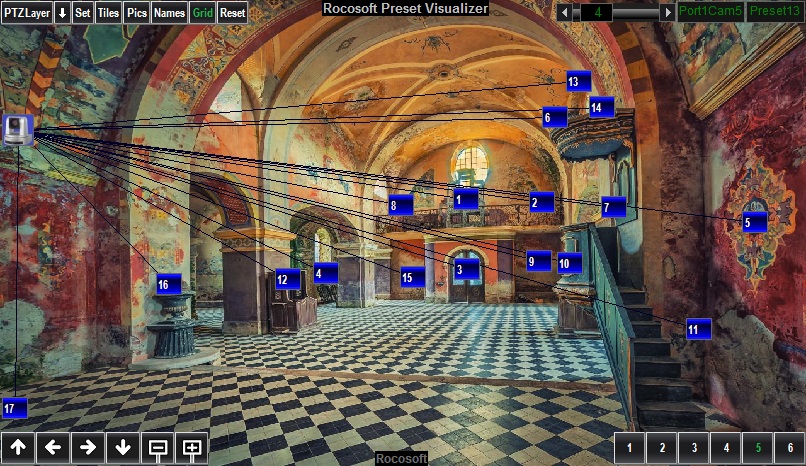The image appears to be a screenshot from a video game set in a grand, historic building, possibly a temple or old church. The scene features a large, open room with several tall, red and brown arches leading into adjacent rooms. The ceiling is intricately designed with arches that create a goldish pattern, including an "X" shape. The floor displays a black and white checkerboard tile pattern. 

On the right-hand side, a few short stairs lead up to an elevated level. The left side has stone walls with tables up against them and noticeable splashes of red, black, and orange, suggesting worn mosaics or paint. Scattered throughout the scene are blue rectangles labeled with numbers from 1 to 17, possibly highlighting specific features.

The bottom of the screen includes interface elements: in the lower left corner, there are arrows (up, side, side, down) next to minus and plus signs, all inside small boxes. The lower right corner displays numbers 1 to 6 in boxes, with the number 5 in green and the rest in white. Across the top of the image, several tabs read "PTZ Layer," "Set," "Tiles," "Picks," "Names," "Grid," and "Reset." The top middle section has a black bar labeled "Rokosoft Preset Visualizer." Additional details include various colors like burgundy, red, orange, yellow, gold, brown, black, and white, enriching the scene's overall historic and ornate aesthetic.